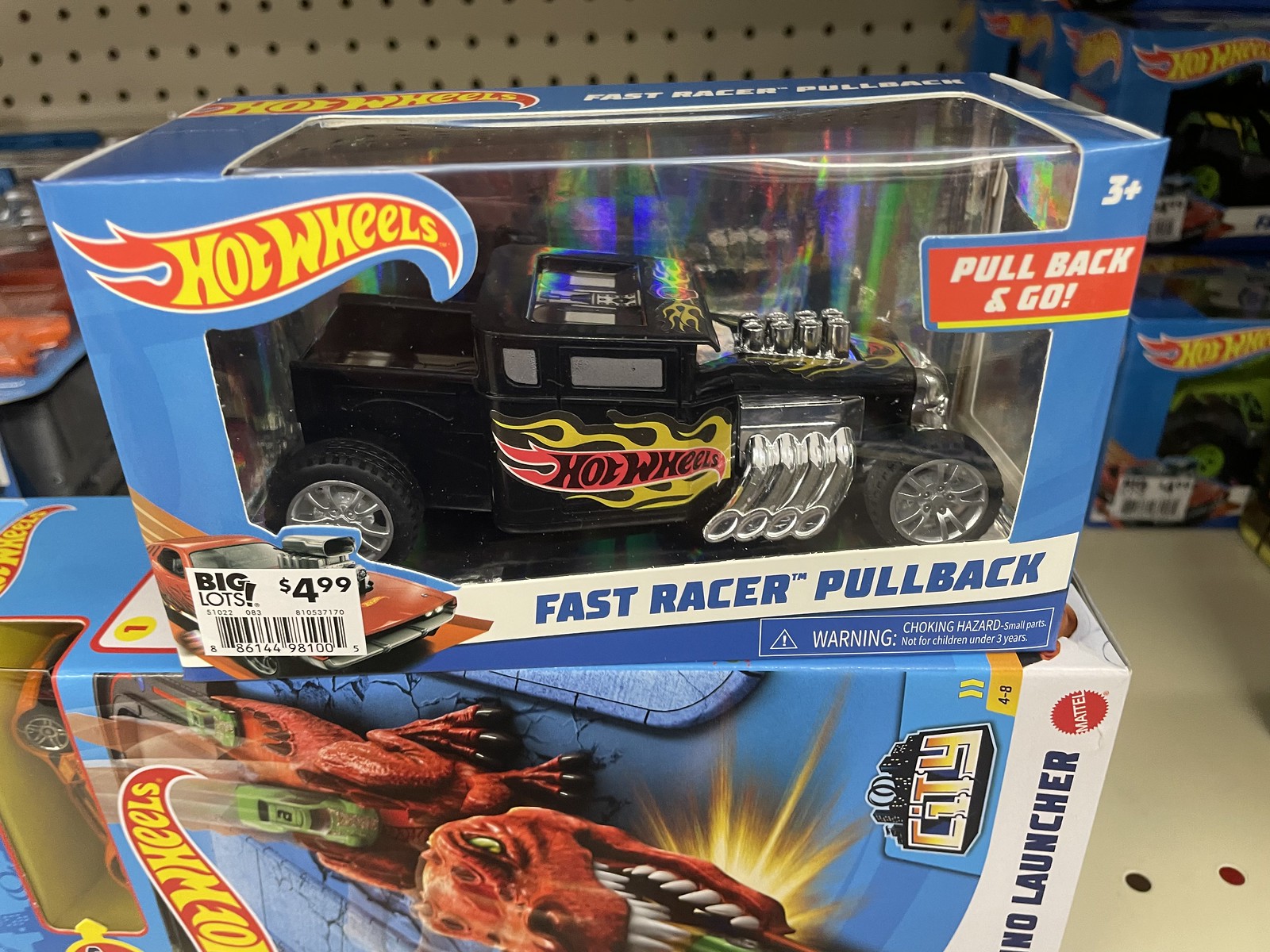The image depicts a display in a toy store, specifically showing a shelf with a grayish-beige pegboard backdrop featuring an evenly spaced series of small holes. On the shelf are two prominently displayed Hot Wheels toy boxes. The bottom box showcases a pterodactyl-like creature with red skin and large white teeth, mouth agape, with "Hot Wheels" emblazoned in yellow text on a red background. The text on the box includes "launcher" in blue letters against a white background. Resting on top of this box, and laid on its side, is another Hot Wheels package that we can see through its clear cellophane front. This box contains a black, old-fashioned hot rod pickup truck with exposed aluminum exhaust pipes and cylinders, no hood, and "Hot Wheels" written across the doors. The packaging also states "pull back and go" on a red background. A small price tag on the left side of this box reads "Big Lots $4.99" with a bar code underneath. The display is not well-lit, casting a few shadows, and giving the impression of varied Hot Wheels models available for sale on the shelves, which might be yellowish-white perforated metal.